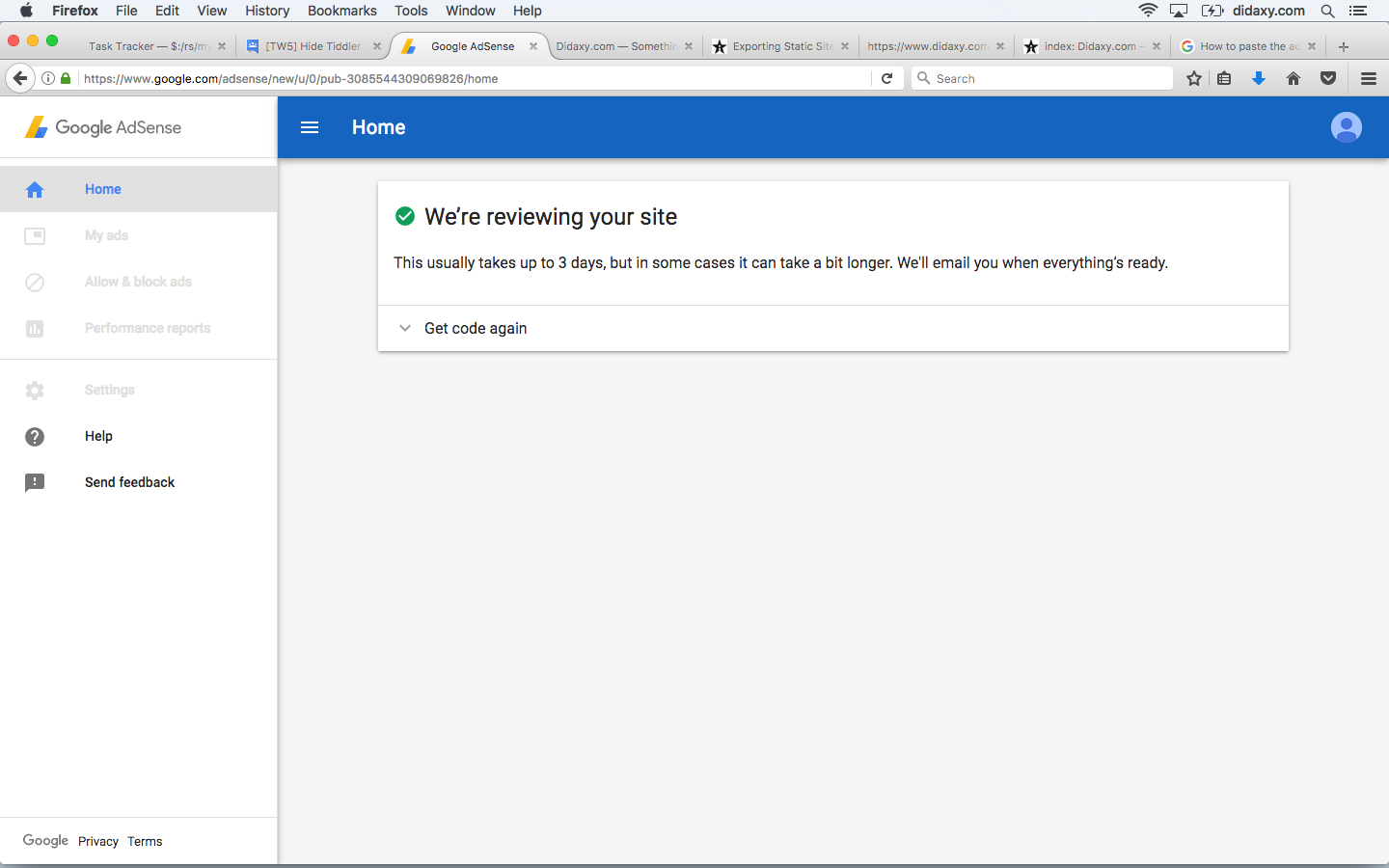This image captures a screenshot from a computer screen. In the upper left corner, the familiar Apple logo indicates that the image is taken on a Mac. Adjacent to it, the menu bar includes standard options such as "Firefox," "File," "Edit," "View," "History," "Bookmarks," "Tools," "Window," and "Help."

On the right side of the menu bar, a signal strength icon is visible, followed by an indistinct icon, and a battery icon indicating that the battery is low and needs charging. Next to these icons, the text "D-I or D-L-D-A-X-Y.com" is partially visible, followed by a search icon and a menu icon represented by three horizontal lines.

The main content of the screen displays the Google AdSense home page. The navigation options "My ads," "Allow and block ads," "Performance reports," and "Settings" are listed but appear grayed out, suggesting they are not clickable. Below these, "Help" and "Send feedback" are visible and appear to be active clickable options.

Centered on the screen is a message indicating the status of the user's site review on Google AdSense. A green circle with a white checkmark inside is accompanied by the text: "We're reviewing your site. This usually takes up to three days, but in some cases, it can take a bit longer. We'll email you when everything's ready." Below this message, a drop-down arrow and the option "Get code again" is available.